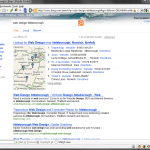The image is a screen capture from a desktop computer, featuring a highly blurred display. The main content appears against a white background. Horizontally positioned black bars frame the top and bottom of the screen. At the very top, the black bar is followed by a web address bar housing various icons. Beneath this, there's a depiction of sky and clouds in dark gray and green hues. The center of the screen contains a series of indiscernible texts interspersed with an image on the left, which vaguely resembles a map. To the right of the map, several lists are present, comprising sentences and words in both blue and black text. Further below, additional information is written in similarly colored text, though the severe blurriness renders this text unreadable.